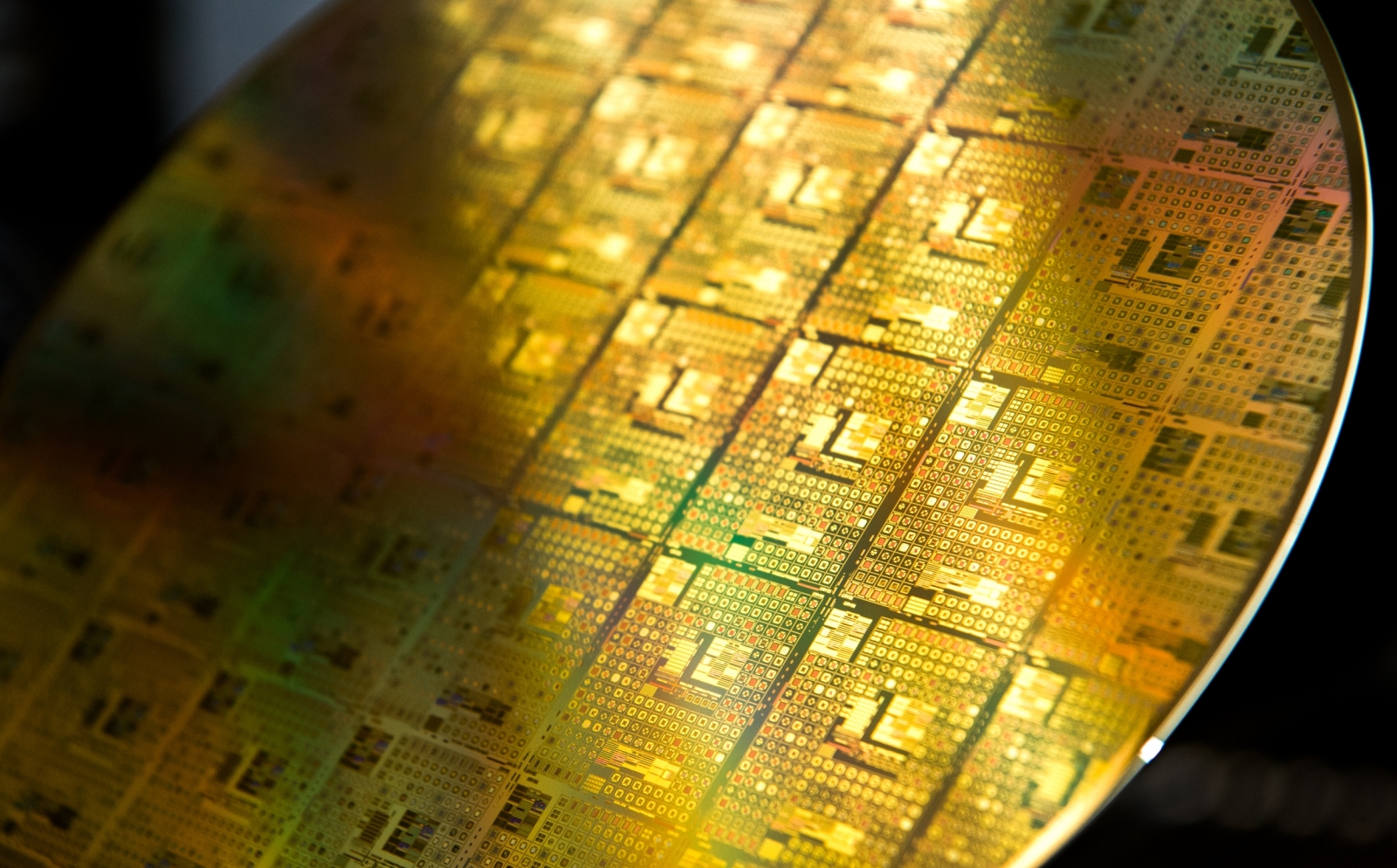This is a highly detailed, full-color close-up photograph of a circular semiconductor chip with a reflective gold surface. Set against a black background, the chip dominates the horizontally rectangular image. The chip features an intricate design composed of numerous square and rectangular elements. Especially prominent are the tiny gold squares that fill each larger square and rectangular section on the chip's surface. The chip is framed by a golden border, and the left and right edges are shaded, making the bright center stand out. In this well-lit central area, there are intricate details like small red and white circles and squares, and patches of green possibly indicating the underlying substrate. The light beautifully highlights the reflective quality of the gold, creating a visually striking contrast between the illuminated center and the more subdued edges.